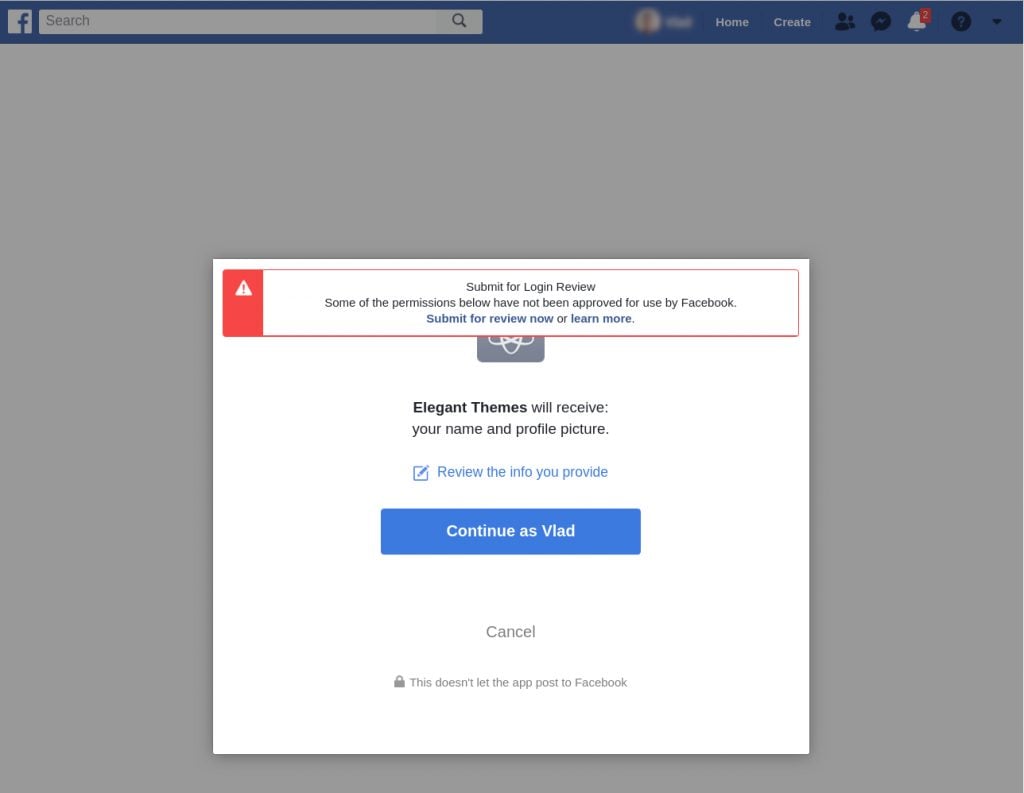Here is the refined and detailed caption:

The image showcases a Facebook page with the familiar blue Facebook banner across the top, featuring the white 'F' in a blue box on the left side, followed by a white search bar. The user's profile picture and name, which have been blurred out for privacy, are also visible. Below this, the navigation bar includes options for 'Home', 'Create', an icon to add friends, the Messenger icon, and a notification bell indicating two new notifications with red markers. A help icon represented by a question mark inside a circle is also present.

The main section of the page is darkened to highlight a pop-up notification appearing in the center. This popup is a white box with a red outline, including a red ribbon running vertically along its left edge. At the top of this box, a red triangle with a white exclamation mark indicates an alert. The header within the box reads in bold text, “Submit for Login Review,” accompanied by a message stating that some permissions have not been approved for use by Facebook. 

The message outlines the steps for submitting the required information, emphasizing the “Submit for Review Now” and “Learn More” options in bright blue text. Below this, it mentions that “Elegant Themes will review your name and profile picture.” The user is prompted to “Review the info you provide” in bright blue text as well. At the bottom of the box, there is a bright blue button that reads “Continue as Vlad” in white text, with an option to "Cancel" directly beneath it.